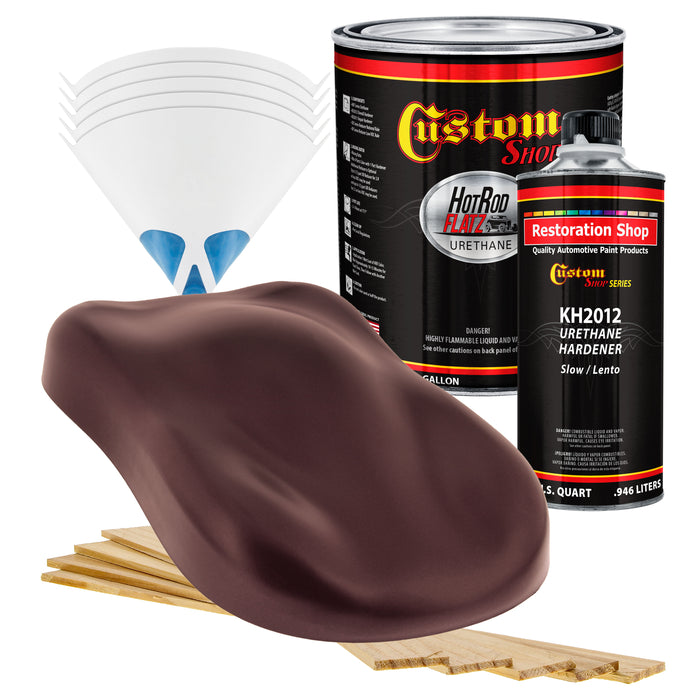The image depicts two distinct cans of automotive paint and hardener on a bright, naturally lit background. The larger can appears to be gallon-sized, predominantly black with red, silver, and yellow accents. It features the text "Custom Shop Hot Rod Flats Urethane" in medieval-style yellow font outlined in red. The smaller can, a vertical one with a black twist cap, is similarly black with red and yellow bands at the top and bottom, labeled "Restoration Shop" and "Custom Shop Series Urethane Hardener" along with "KH2012 Urethane Hardener Slow/Lento." Both cans exhibit a metallic silver top. In the image's periphery, there are clear plastic funnels with blue accents, light-colored wooden paint mixers, and what appears to be a dusky purple object reminiscent of a tongue against light planks of wood, with white cones stacked in the background. The details are sharp and clearly visible, contributing to a well-lit and vivid presentation.